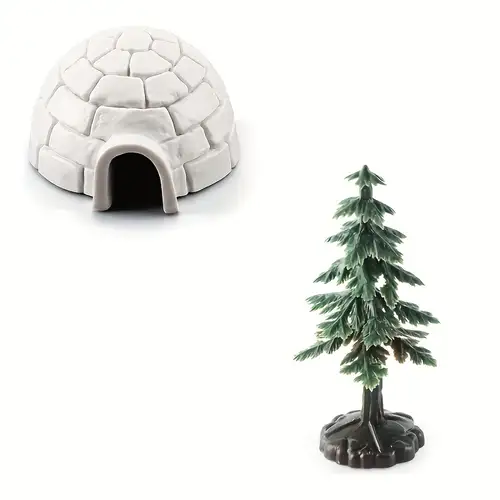The image depicts a square, approximately four-inch by four-inch, with a very light background that can be perceived as either light peach or nearly white. Positioned in the upper left-hand corner is a toy model of an igloo, featuring a white, dome-shaped structure with an arch-shaped, U-like opening at the front that appears black inside. The igloo is constructed with five layers of stacked ice blocks, topped with a single capstone completing the sixth layer. In the lower right-hand corner stands a plastic evergreen tree, with branches tipped in white or silver, suggesting snow. The tree has a brown trunk and a round, dark brown base that includes visible roots and rocks, enhancing its realistic appearance. The objects seem to be 3D models or toys, adding a decorative element to the image.